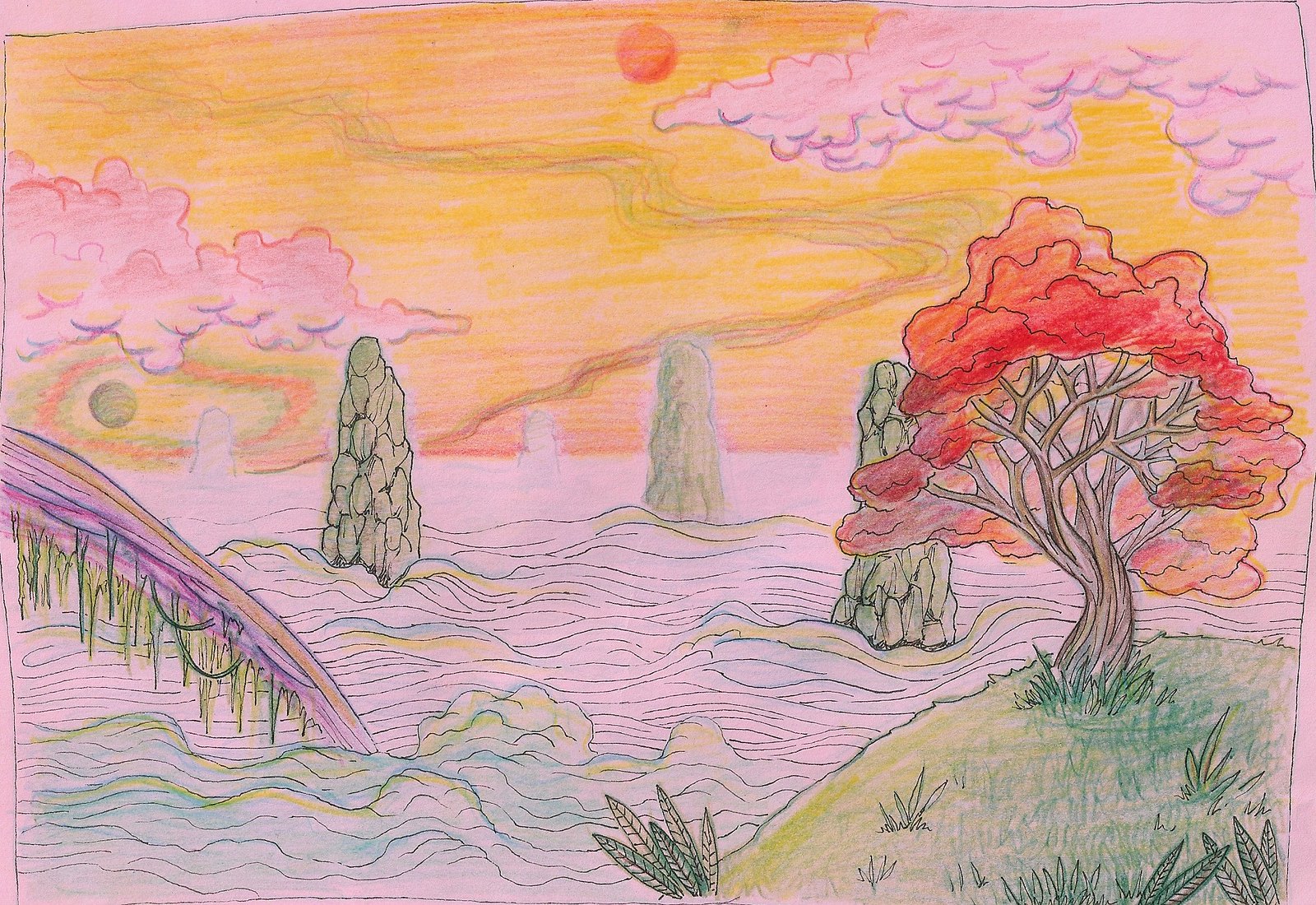This vibrant, hand-drawn artwork captures a picturesque, fantasy-inspired landscape. In the foreground on the right, there's a verdantly colored hill adorned with an intricately twisted tree. The tree's branches, sprawling elegantly, are laden with a mix of red, orange, light pink, and purple foliage. Surrounding the hill, various green blades of grass and small plants add to the lushness of the scene. To the left, patterns of waves hint at a body of water in shades of white, light gray, and accented with soft blue and yellow hues. Above these elements rise tall, green-shaded rock formations, their peaks partially shrouded, enhancing the mysterious atmosphere. Occupying the background is a vivid sky, transitioning from orange to yellow, adorned with drifting, pink-outlined clouds. Prominently featured is a singular red circle in the upper center, suggesting a sun or moon. A streak of colors described as a rainbow with vines – one line yellow, another purple with green accents – adds a whimsical touch to the pastoral scenery. This detailed depiction provides a very pleasant and dreamlike environmental space, expertly illustrated with what appears to be colored pencils on a white canvas or art paper.